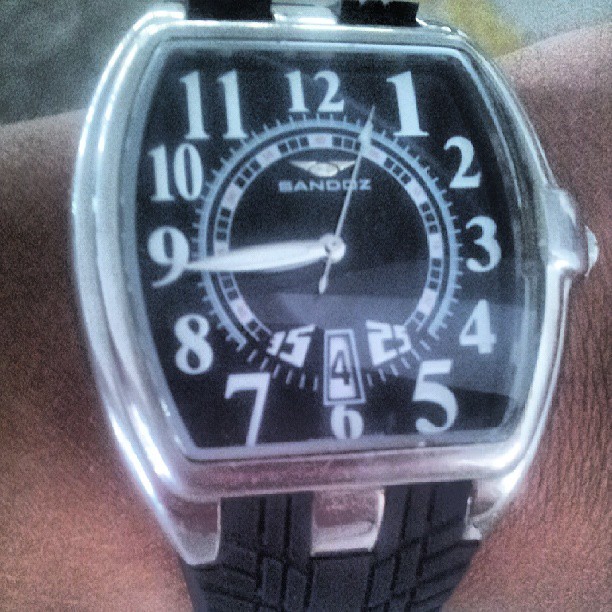This photograph captures a close-up of a wristwatch on a person’s brown-toned wrist. The analog watch features a distinct black band with a pattern resembling tire treads and a shiny silver metal case. The face of the watch displays numerals 1, 5, 7, and 11 enlarged and in white, while the other numbers are uniformly smaller. The hands of the watch — the minute, hour, and second hands — are also white, with the second hand currently at the 3-second mark. The time reads approximately 9:44, just before quarter to ten. Positioned below a silver wing emblem in the center is the brand name "Sandoz." The watch's face includes additional elements: on the left, the number 35 in white, on the right, the number 25, and a small triangle with the date "4" in black on a white background. A circle with small squares around its perimeter also adorns the watch face.